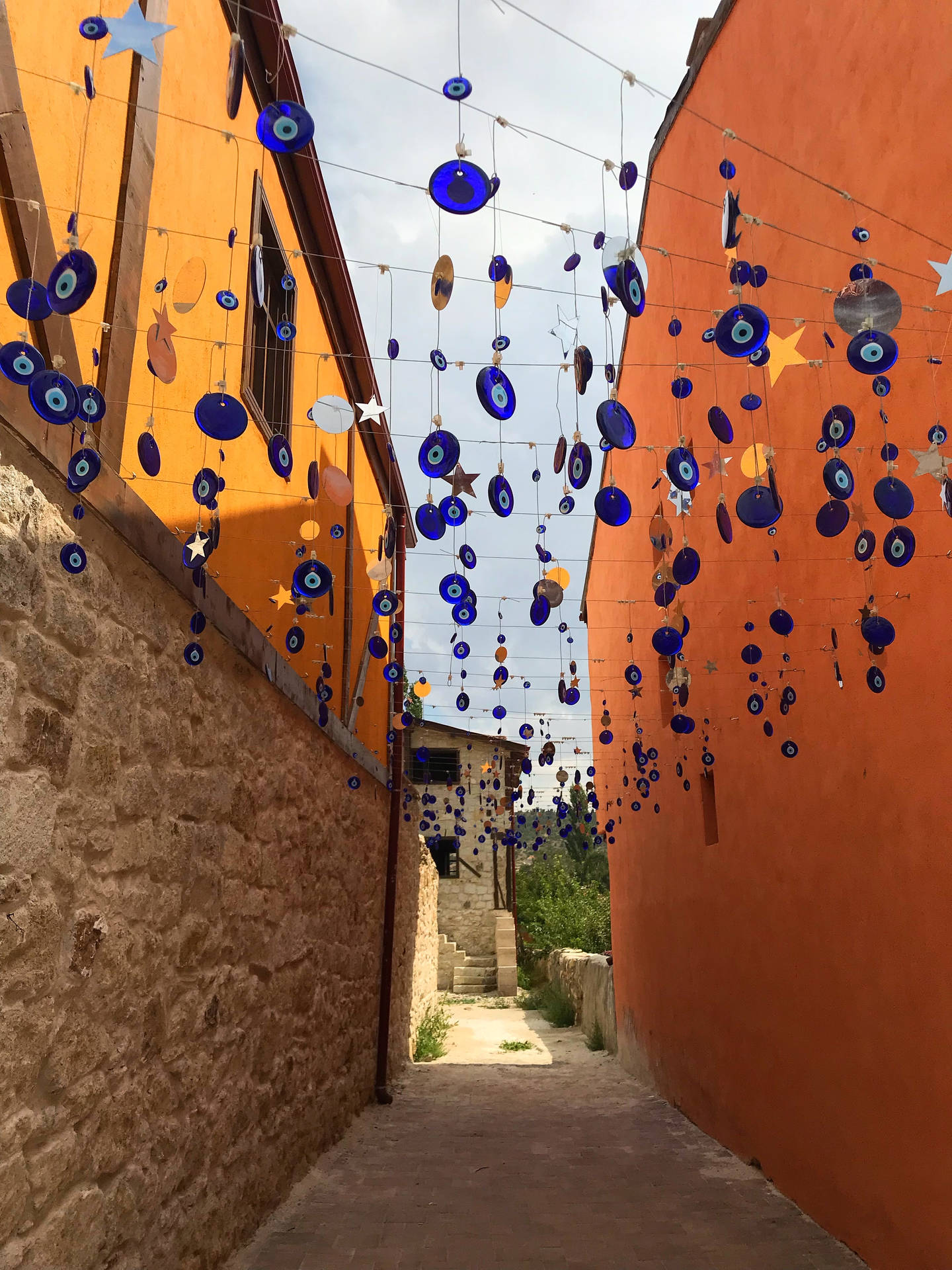This is a detailed outdoor daytime photograph of a colorful Mediterranean-style alleyway. The alleyway is framed by two rustic buildings approximately two meters apart. On the left, the lower half of the building consists of wide blocks of lightly cemented stone, while the upper half features vibrant yellow plasterwork with dark brown beams and a central framed window. The right building has a solid burnt orange plaster wall with a few small cut-out windows. 

A striking feature of this scene is the array of hanging objects strung across numerous wires between the buildings. These objects include hundreds of blue glass pendants depicting traditional evil eye wards, characterized by their dark blue outer ring, lighter blue inner circle, and central black pupil. Complementing these are gold and silver reflective stars and circles. The hanging decorations, swaying in the breeze, create a mesmerizing effect under the sunny sky dotted with white clouds.

At the end of the alleyway stands a small stone shack with steps leading up to it, appearing somewhat in disrepair and likely uninhabited. To its right is a lush green bush, framing the rustic scene. The overall atmosphere exudes a charming, sunlit Mediterranean or Turkish ambiance, with a mix of bright colors and traditional decorative elements.